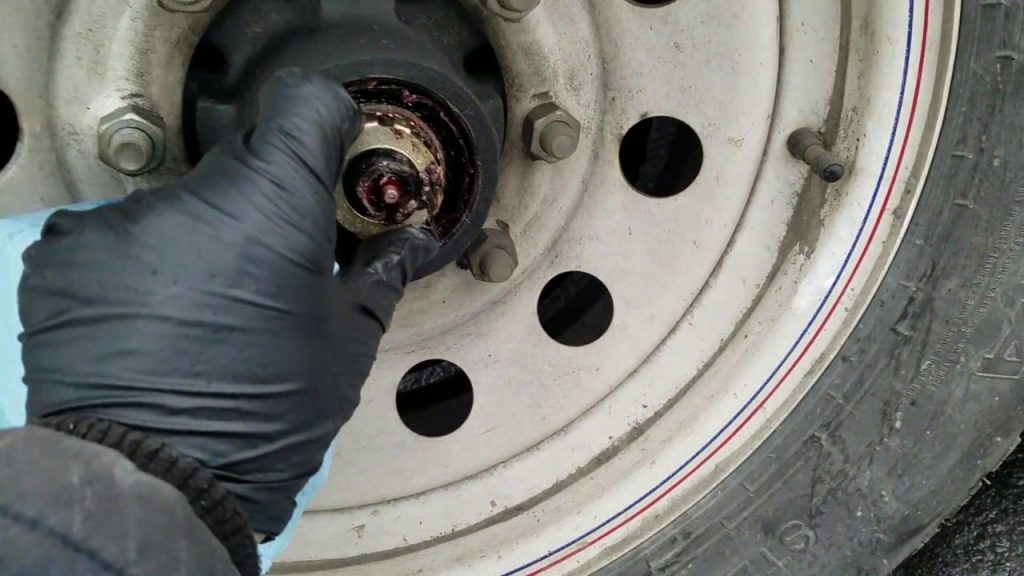A detailed and up-close photograph of a vehicle's tire is depicted here. The image is centered on the bottom middle portion of the tire, which extends upwards and off to the top right edge, about an inch from the right side. The rim's edge is visible, featuring a striking combination of colors: a white border, followed by a thin red line, then about a quarter to half an inch of gray, succeeded by thin blue and more white moving inward.

From the bottom left corner, a person's wrist and hand are visible, clad in a black coat and glove. The gloved hand's pointer and middle fingers reach out to grasp the wheel's center. The wheel's hub is silver with a black center and a black surrounding edge, encircled by lug nuts. There are small holes arranged around the rim: three along the right side and one on the partially visible left side.

From the right corner, a section of the black tire extends downwards to around two inches from the bottom right, then angles leftward to a similar distance. The tire appears quite worn, displaying lighter patches that fade to gray. At the bottom, a portion of the tread is visible, showing letters "S" and "T." The bottom right corner of the image reveals a black surface, likely the concrete ground.